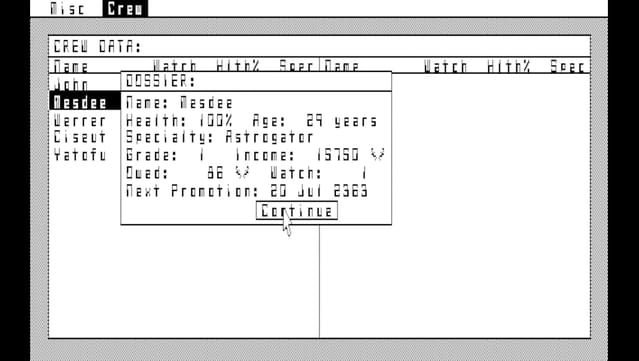The image depicts a low-quality, black-and-white screenshot from a retro-futuristic computer interface. The pop-up box labeled "dossier" showcases detailed crew data, specifically for an individual named Macedo. This includes information such as their health status (100%), age (29 years old), specialty (astrogator), grade (one), income (157.90 quad), watch (eighty-six), and the date of their next promotion (July 20th, 2363). The interface design mimics old computers from the 1970s and 1980s, like the Commodore 64 or early Apple models. The screen also displays hierarchical crew positions, with more details appearing when Macedo is selected. The mouse pointer is blurred but visibly hovering over the "Continue" button, accentuating the era-specific and cinematic aesthetic of this fictional computer system.